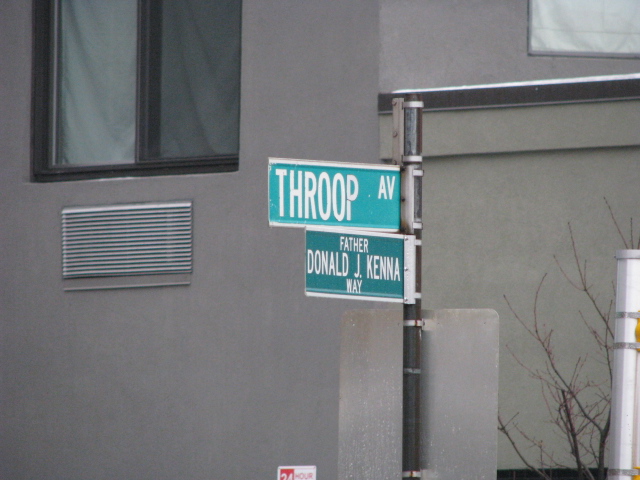This photograph, taken outdoors, predominantly features the exterior of a dark gray building that transitions to a lighter gray towards the bottom and side. Central to the image is a street sign on a black metal pole, attached by silver clasps to two green rectangular signs with white borders. The top sign reads "THROOP AV" and the lower one, pointing left, reads "Father Donald J. Kennaway." In the background, there's a large, rectangular window with a black wooden frame, draped with white curtains. Beneath the window, on the left side, is a white rectangular air conditioning vent supported by a dark gray base. Another partially visible window on the right is also adorned with white curtains. An intriguing element in the image is the portion of a leafless tree with dark brown, light brown, and red accents on its branches. Additionally, there's a small white box and the back of a silver sign, both cut off at the edges. Lastly, a secondary white sign next to the street sign pole is partially readable with the number "24" and some red text.